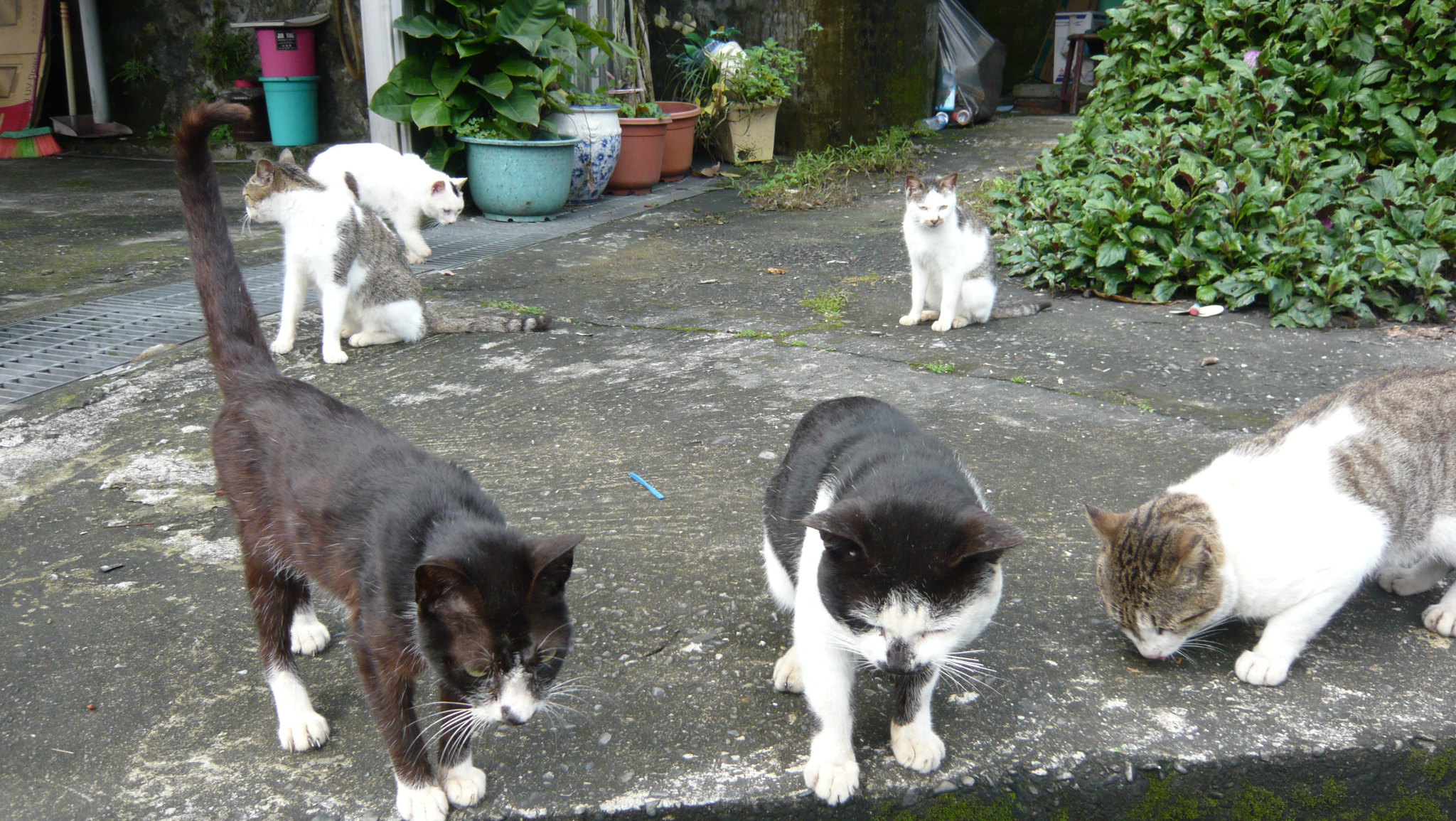This photograph, likely taken in someone's backyard or driveway, captures a charming scene featuring six cats amidst a variety of elements. The setting includes a wet concrete patio, suggesting it recently rained, with a large green bush boasting bright green leaves in the top right corner. Spread across the upper frame are various flower pots — two red, one white, and one teal, along with additional terracotta, ceramic, and a square plastic pot. Accompanying these are items like buckets, a dustpan, a broom, and plastic bags, suggesting a lived-in, outdoor area, possibly near a garage.

At the center of the image, the main subjects are six cats interacting near a dark grey stone slab. In the foreground, three cats are closer to the camera: 
1. A leftmost brown cat with a white nose and paws, standing alert with its tail extended upwards.
2. A middle black cat with a predominantly white body and face, also with white legs, seemingly focused on the ground.
3. A rightmost cat, displaying a mix of tabby stripes and white fur, appears to be engrossed in something on the concrete.

Further back, additional feline figures comprise:
1. A predominantly white cat with a patch of black on its head, situated nearest to the flower pots.
2. A grey and white cat, mirroring the patterns of its surrounding companions, positioned slightly behind the first black cat.
3. Another grey and white cat closer to the green bush, sitting serenely.

The cats display various behaviors, from sniffing the ground to sitting and gazing around, adding a dynamic feel to the tranquil, leafy setting.